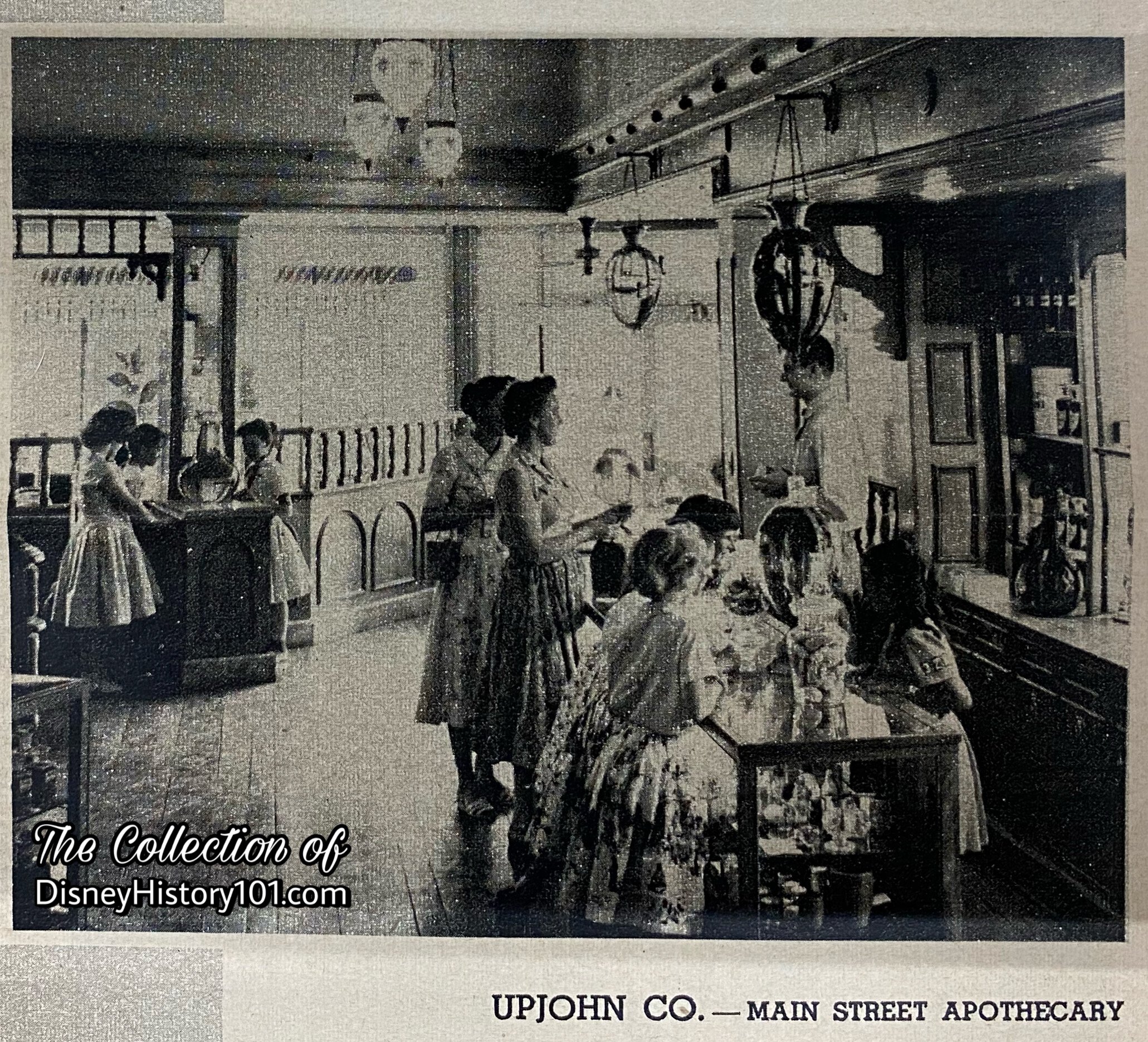This black and white vintage photo, seemingly printed in a newspaper, showcases the Upjohn Co. Main Street Apothecary. The image is part of the "Collection of Disney History 101.com" as noted on the left side. The scene captures a lively business, likely a place where customers would come to enjoy sodas and sweets. Two women, dressed in period attire, are engaged in conversation with a man standing behind a counter adorned with an assortment of sweets. To the right of them, three children—two in front of the counter and one behind—adorned in dresses, are eagerly eyeing the array of confections stored in glass jars. On the left, another woman stands with two children who are intently examining a different jar of sweets on a separate table. The building features an abundance of windows at the front, allowing light to illuminate the wooden floor, adding to the nostalgic ambiance of the apothecary.